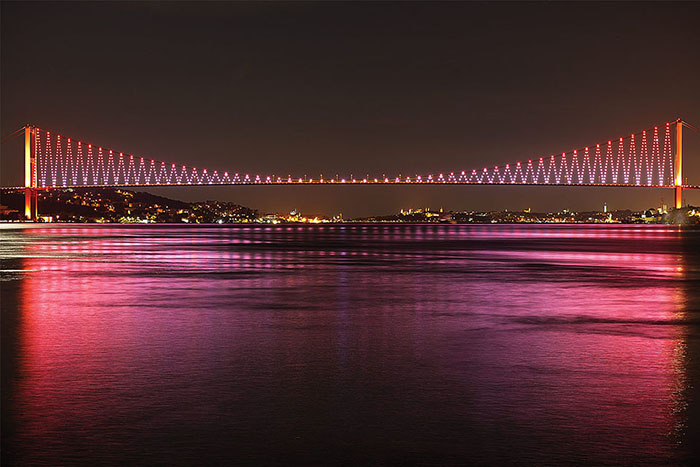A nighttime photograph captures a vast, illuminated bridge spanning over a body of water, with a bustling cityscape and hilly areas visible in the distant background. The bridge, distinctly prominent against the dark sky, features a unique architectural design where the supports rise at each end and gracefully descend towards the middle, forming a bow-like shape. The structure is adorned with vibrant, pinkish-yellow lights that trace symmetrical triangular patterns along the length of the bridge, resembling festive decorations. These striking lights reflect vividly on the water below, casting a mesmerizing pink glow that dominates the scene, surpassing even the city's twinkling lights in luminance.